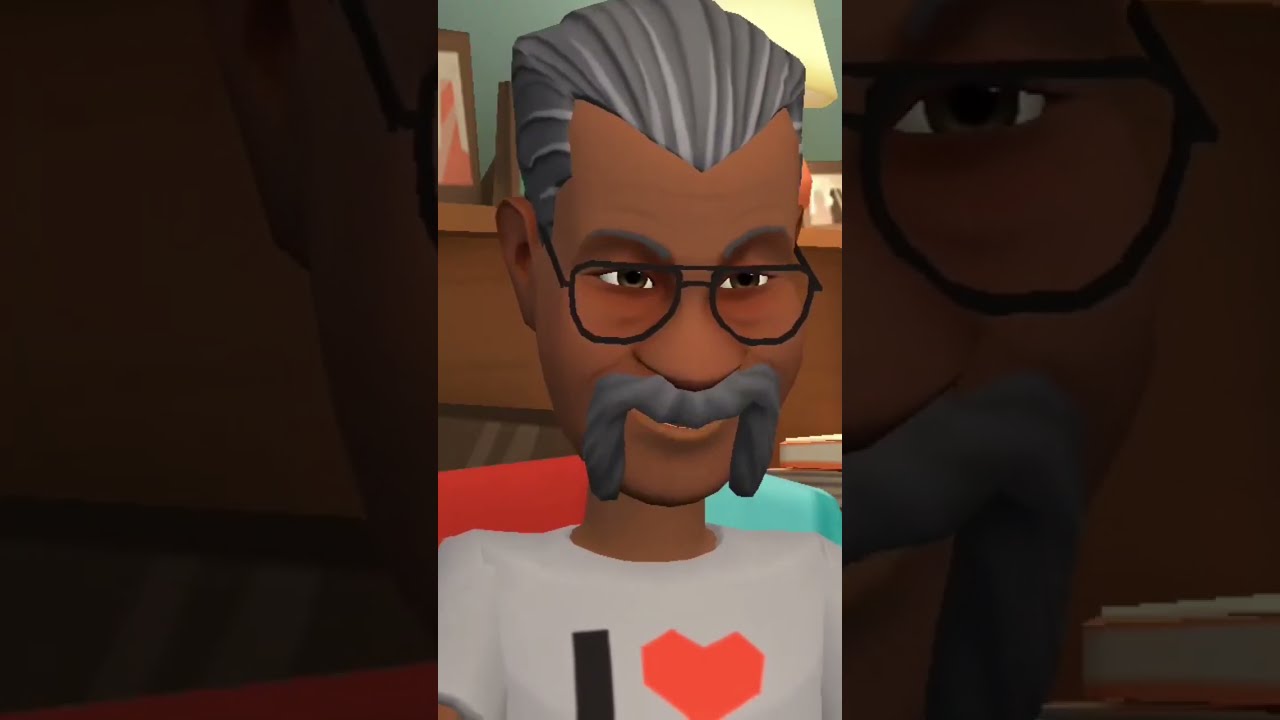The image is a rectangular, six inches wide by three inches tall, featuring a detailed caricature of an older African-American man positioned at the center. The character has distinct gray hair with a prominent widow's peak, a handlebar mustache, and wears black-framed glasses resembling aviators. His expression appears focused, looking downward. He sports a white t-shirt displaying a black "I" followed by a red heart, though the rest of the text on the shirt is obscured.

Behind the central character, a brown mantle adorned with pictures is visible, indicating a domestic setting. The character sits in a blue chair with a red blanket draped over one side. On the left and right sides of the central image are enlarged, darkened close-ups of the man's face. The left side highlights his ear and part of his glasses, while the right side showcases his eye and handlebar mustache, creating a cohesive yet dynamic portrait. The overall style suggests a cartoon or a video game avatar, with a focus on vibrant yet muted hues including white, black, red, pink, gray, brown, and yellow, and a distinct polygonal, low-quality texture indicative of a mobile app or video game screenshot.